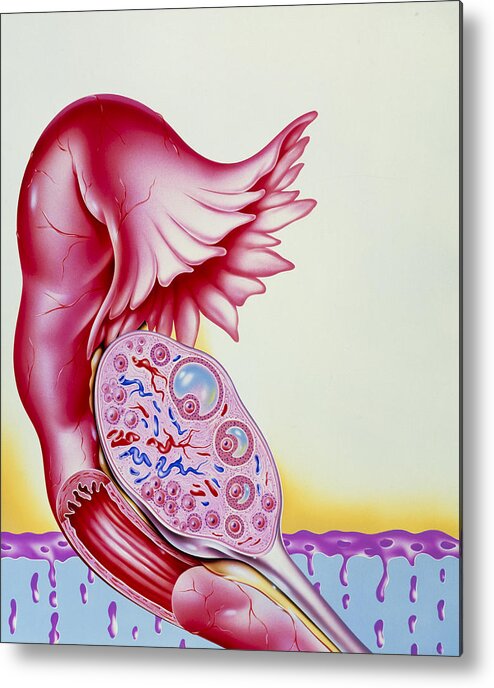In this detailed cartoon image, the central focus is a depiction of the fallopian tube and ovary against a predominantly yellow background, transitioning into shades of aqua blue and purple at the bottom. The fallopian tubes, which curve upward before descending, are illustrated in a reddish-pink color and feature fimbriae, finger-like projections, reaching toward the ovary. The ovary itself is a pinker hue and includes red and blue squiggles that represent arteries and veins. Nestled inside the ovary are multiple circles symbolizing eggs, progressively increasing in size to indicate growing follicles.

Some interpretive elements add a fantastical dimension to the anatomical illustration, with the overall shape resembling a creature or flower breaking through soil-like substance colored in aqua blue and purple. Additionally, elements of the picture, including pink and blue circles and lines and large tube-like blooms, evoke a sense of a creature with a pair of eyes or an open mouth, further blending organic and biological motifs. This combination of detailed anatomical accuracy with imaginative, almost surreal features creates a multifaceted and fascinating image.